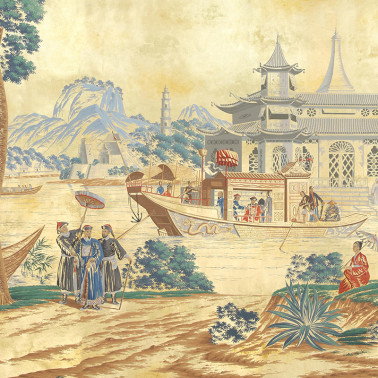The painting depicts an idyllic scene from what appears to be feudal Japan, rendered in soft, light watercolors. Dominating the scene is a large, tranquil river or lake where a boat glides gracefully, manned by two individuals working the oars while several others, dressed in blue, red, and black attire, enjoy a leisurely cruise. Surrounding the boat, the landscape unfolds with meticulous detail: a grand, traditional Japanese temple with elegant doors and arches stands prominently to the right, its pristine white walls contrasting with the natural elements.

In the background, a majestic mountain dotted with trees and hints of blue and white shades—possibly snow-capped—dominates the horizon, blending into the light brown sky. Near the temple and extending towards the side of the painting is a tall, white tower, adding to the architectural splendor of the scene.

In the foreground, a mud embankment and path are populated with figures engaged in various activities. On the left, several people dressed in black and blue robes carry wooden umbrellas, while to the right, a woman in a striking red robe sits alone, possibly lost in thought. Scattered green shrubs and trees punctuate the otherwise earthy tones of the ground, adding a touch of greenery that further enhances the serene atmosphere of this historical vista.